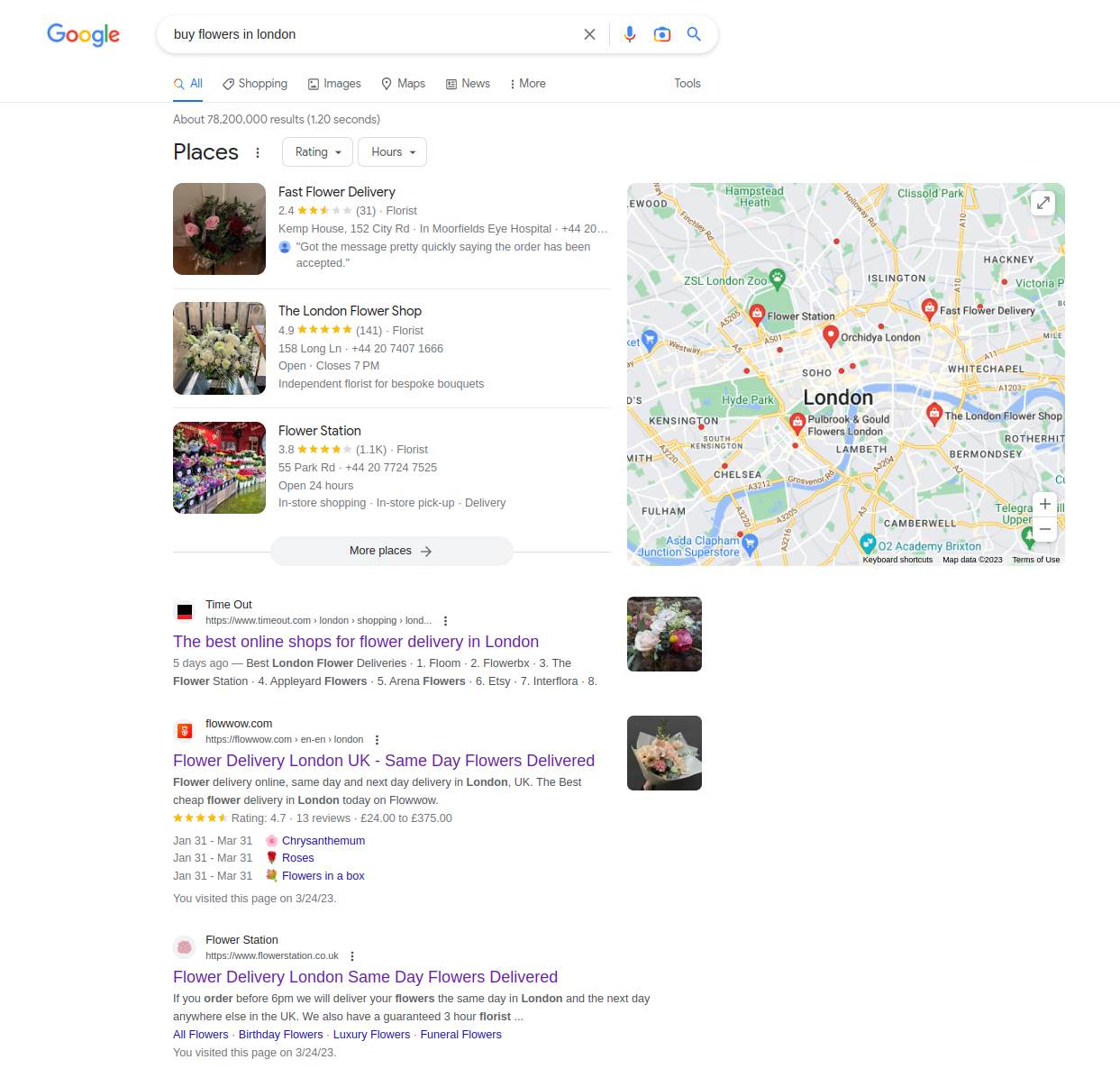The image displays a Google search results page. At the top left corner, the Google logo is prominently featured. Below it, within the search bar, the query "buy flowers in London" is typed in black text. The main results page shows three highlighted flower shops, each with pictures on the left, followed by their distance, ratings, and brief descriptions.

1. The first shop listed is "Fast Flower Delivery".
2. The second shop is "The London Flower Shop".
3. The third shop is "The Flower Station".

To the right of these listings, a map of London is visible, with each flower shop pinpointed. The map is a square segment of London, showcasing the exact locations of these shops.

Below the specific store listings, additional search results are displayed. The first option is "More places", followed by "The best online shops for flower delivery in London", "Flower Delivery London UK, same day flowers delivered", and "Flower Delivery London, same day flowers delivered". These additional search results offer more choices below the highlighted flower shop listings.